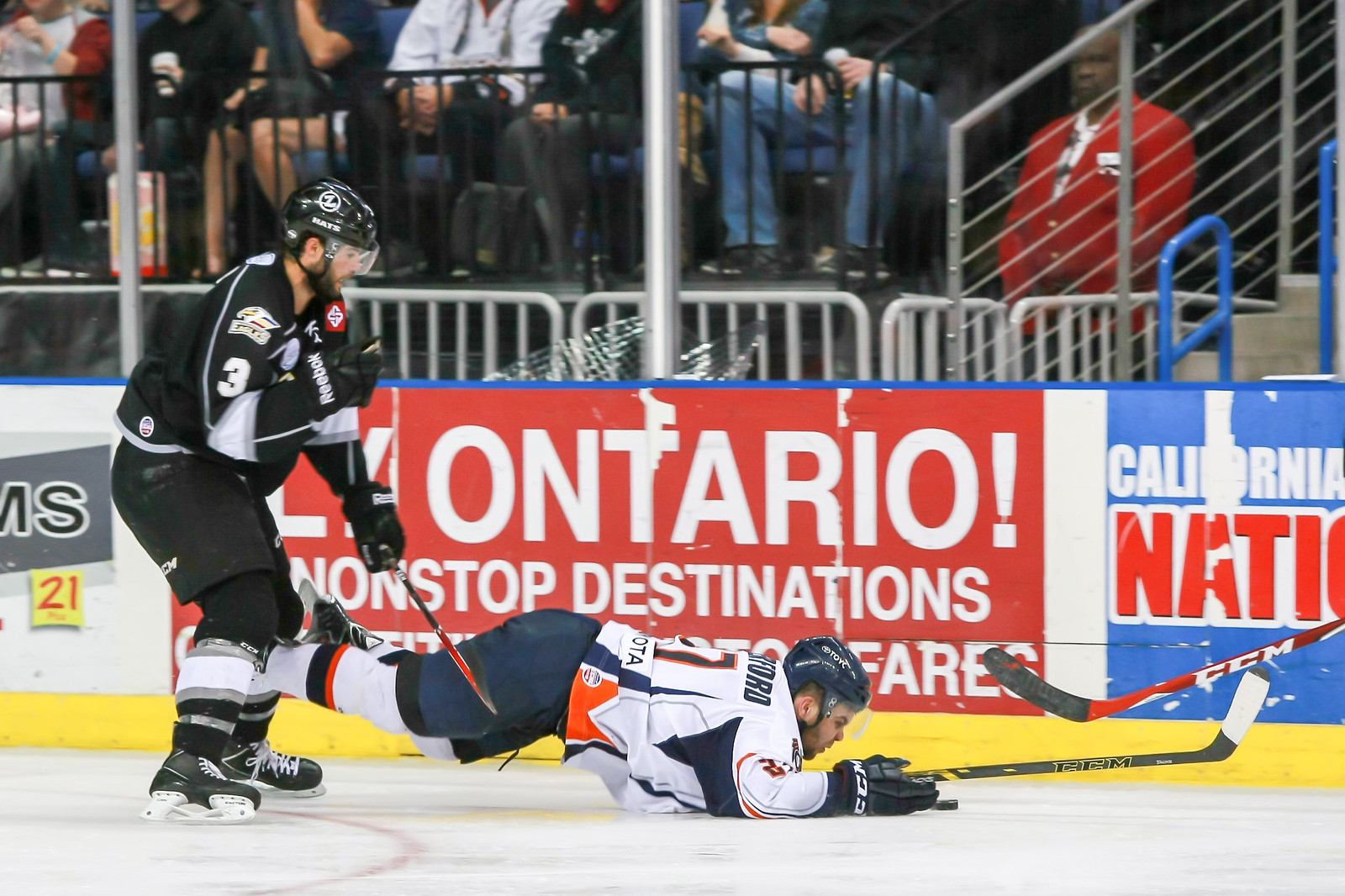In this image captured during a professional hockey game, two players dominate the frame. The player on the left stands upright, clad in a black jersey with white letters, holding his hockey stick poised in front of him. He wears a helmet and appears focused. Directly in front of him, a second player in a blue, white, and orange jersey tumbles onto the ice. His elbows rest on the ice as his legs and knees are in mid-fall, and his stick extends upward in front of him. Both players are Caucasian. To the right edge of the frame, a red hockey stick intrudes, seemingly held by an unseen third player. The ice beneath them is pristine white, characteristic of a well-maintained rink. Beyond the players, the rink is bordered by ad boards. One of these ads, in white print over a red backdrop, reads "Ontario! Nonstop destinations," while another blue sign on the left mentions "California Nationals." A metal barrier separates the rink from the spectators, where several fans are seated with only their legs and arms visible, as their heads are cropped out of the image. In the background, an usher, a black male in a red button-up sweater or sport coat, stands to the right, contributing to the bustling yet organized atmosphere of the event.